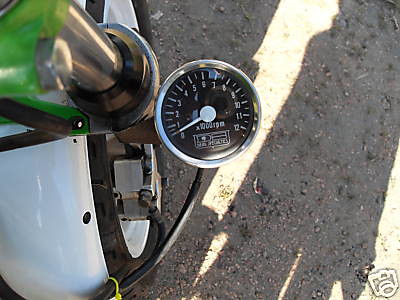The photograph features a pressure or tire gauge prominently displayed against a backdrop of heavy machinery. On the left side of the image, a piece of industrial equipment, constructed from white-painted metal, occupies the space. This machinery includes a substantial steel pole from which the gauge is suspended. The ground beneath the setup is a compacted earthy surface, barren and strewn with rocks, with no signs of grass or vegetation.

To the right, the ground continues to dominate the scene, devoid of any significant features apart from the rocky terrain. The photograph was taken under bright sunlight, casting conspicuous shadows. The shadow of the photographer extends across the ground, alongside the elongated shadows of the machinery, effectively reducing the illuminated areas.

The gauge itself is inactive, with the needle positioned at zero. It is a circular instrument with a black face, embellished with white numerals and markings indicating the measurement range. Encased in silver-colored metal, the gauge reads from zero to twelve, with the number six prominently placed at the apex. A closer inspection reveals an inscription indicating the measurement unit: times 10,000 RPM, confirming that the gauge is designed to measure rotations per minute.